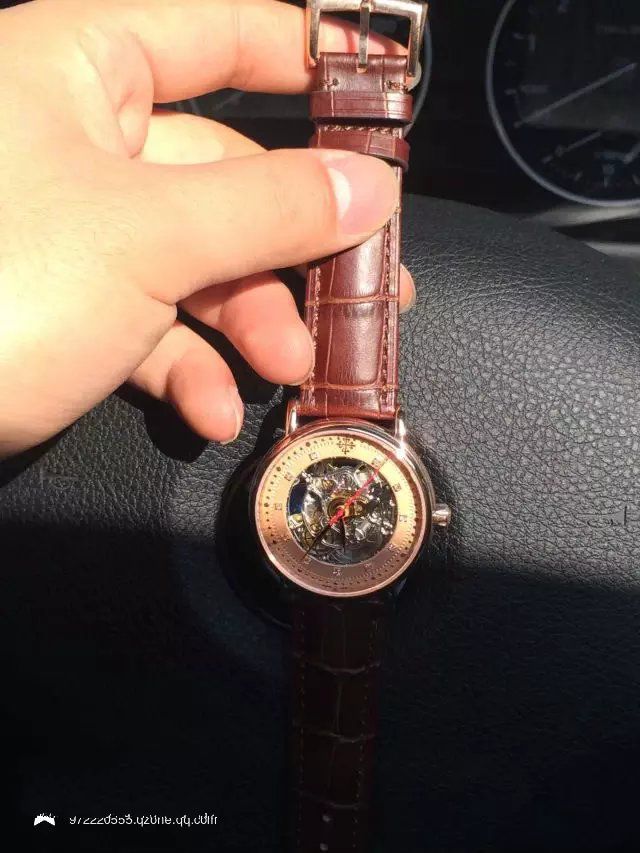This color photograph features a close-up of a wristwatch held by a person's left hand against the black vinyl dashboard of a vehicle. The watch has a brown leather strap with silver buckles and a round face that is beige in color, surrounded by a dark inner rim. Adorned with small, box-like characters instead of traditional numerals, the watch's face includes an intriguing black and white pattern and what appears to be a mass of liquid metal where you'd typically find the gears. The red hands are faintly visible and a silver-colored dial for adjusting the time is situated on the right side of the watch. The background reveals a black steering wheel with a horn logo embossed on the right, and an instrument cluster or gauge just barely visible in the top right corner of the image. Additionally, the bottom left corner of the photograph displays white text and a small logo, likely a website address, though it's too small to read clearly.